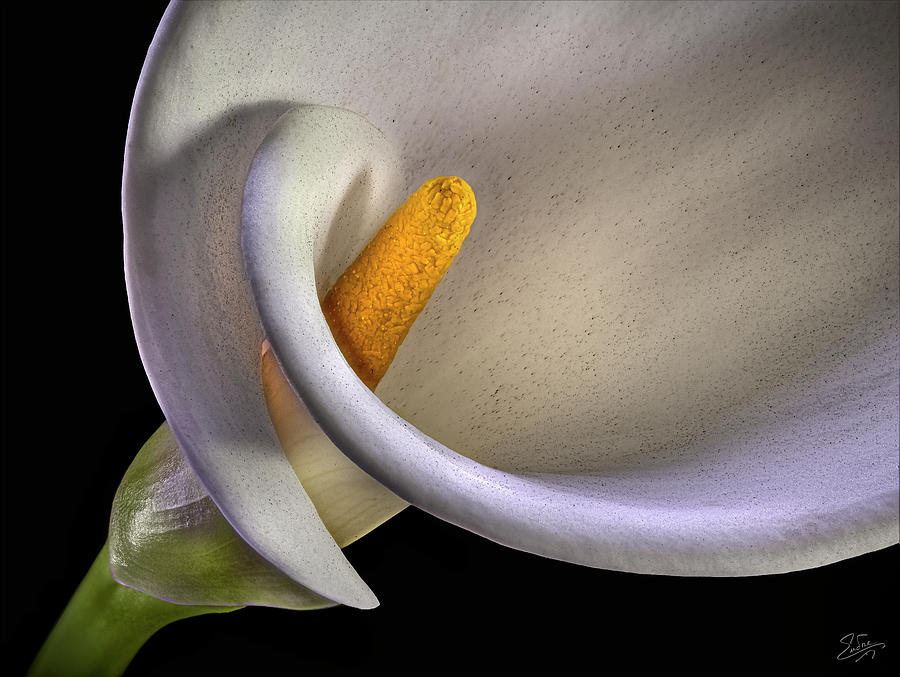This photograph captures an extreme close-up of a calla lily flower, rendered in exquisite detail. The white petal forms a graceful, curly bulb shape that seamlessly transitions into a vibrant green stem visible in the bottom left corner. Central to the image, a prominent yellow pistil rises vividly from the cup-like center of the flower, its hue a striking gold with an almost orange tint. The meticulous depiction suggests this might be a hyper-realistic artwork rather than a straightforward photograph, reinforced by a delicate, hand-drawn signature in the bottom right corner. The flower stands out starkly against a pure black background, emphasizing its flawless, unblemished beauty.